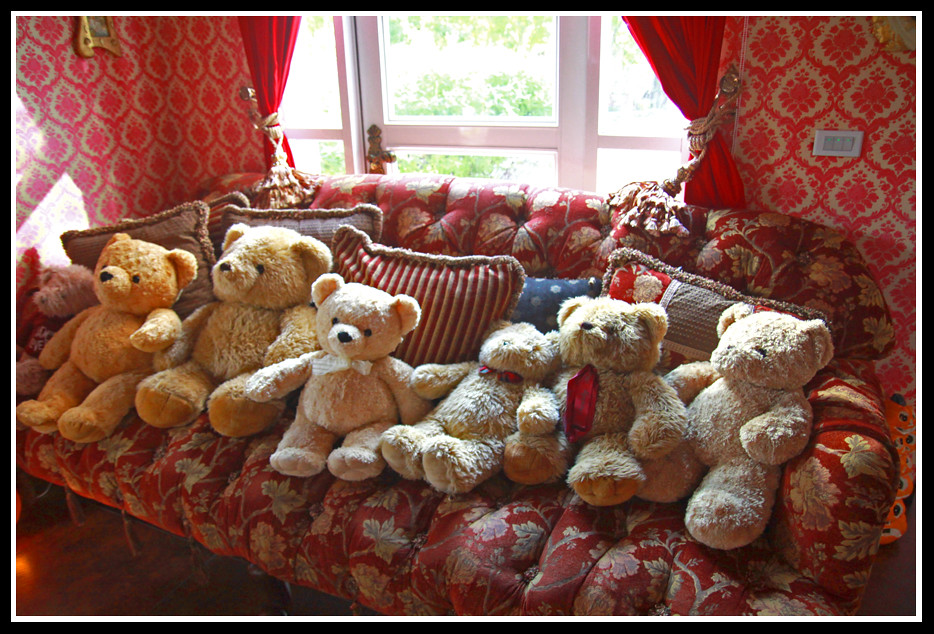In the brightly lit room, the focal point is a striking red couch adorned with an intricate pattern of silver leaves. This couch is home to an assembly of six large, fluffy teddy bears, ranging in hues from beige to apricot. Some bears sport red or white bow ties, with one donning a red shirt. They rest against an array of eclectic pillows, including patchwork, red and silver striped, and blue decorated cushions, adding to the charming scene.

The room features red flocked wallpaper with teardrop-shaped yellow designs, perfectly complementing the red drapes pulled back with gold ties. Behind the couch, a large window allows sunlight to flood the space, illuminating the green foliage of tall trees and bushes outside, suggesting a beautiful day. The window's sunshine glare softens the overall warmth of the room, creating a cozy, inviting atmosphere.